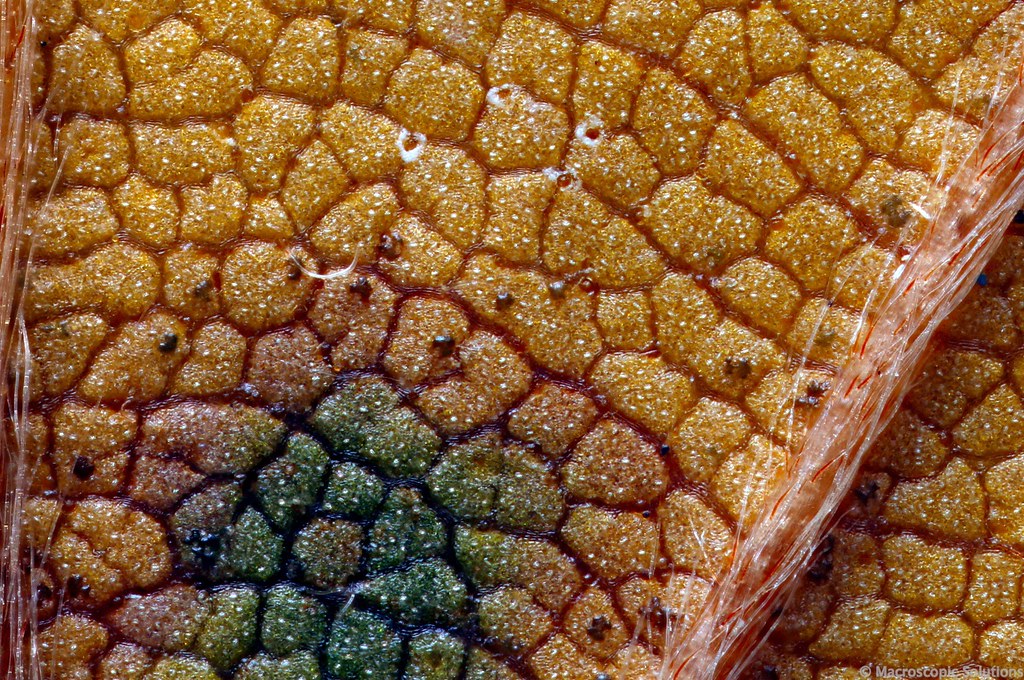The image depicts a zoomed-in, highly detailed view of an unknown organic structure, reminiscent of the underside of a starfish due to its bumpy and crystallized appearance. The central area of the image features vibrant orange, golden, and yellow hues, gradually transitioning towards red, purple, and green as you move outwards. Scattered throughout are fibrous strands that are white and orange, adding to the intricate texture. The surface is covered with numerous tiny, somewhat square shapes, closely packed together, giving the impression of a skin or rock-like texture. Small black specks are visible, possibly indicating minuscule bugs or other elements. Towards the bottom left, the colors shift to a darker, bluish-green, while pink threads can be seen stretching from the bottom right to the top right. The bottom right corner of the image contains a watermark reading "Microscopal Solutions," confirming its likely scientific or microscopic nature.